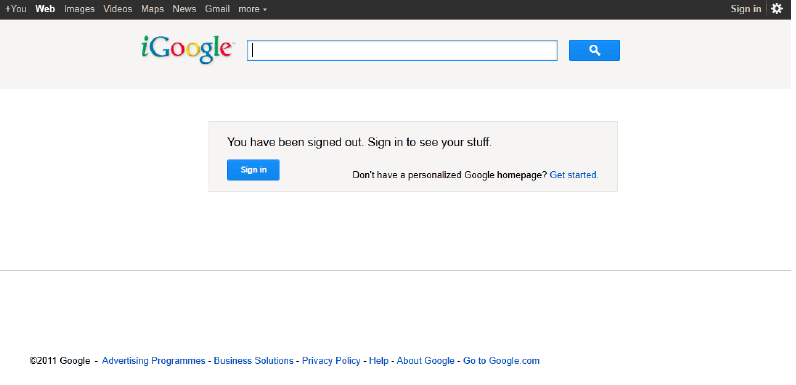This image is a screenshot of the Google homepage from the early 2010s, displayed on a computer screen. The topmost portion, roughly the upper 5%, features a black navigation bar with white text, listing options such as "You," "Web," "Images," "Videos," "Maps," "News," "Gmail," and "More." To the right of these options, there are additional links for "Sign in" and a settings gear icon.

Directly below the navigation bar, the classic Google logo is prominently displayed in its iconic alternating colors of green, blue, red, and yellow. Below the logo, a search box with a blinking cursor is centrally positioned, with a blue "Search" button featuring a white search icon situated to its right.

Further down, the screen displays a message in black text stating, "You have been signed out. Sign in to see your stuff." Beneath this message, there is a blue "Sign in" button. Adjacent to this, another line of text in black mentions, "Don't have a personalized Google homepage?" with a clickable hyperlink labeled "Get started."

The bottom two-thirds of the image contain a thin gray line that separates the main content from the footer. In the footer, positioned at the very bottom of the image, it states "Copyright 2011, Google." Also included are multiple hyperlinks, reading "Advertising Programs," "Business Solutions," "Privacy Policy," "Help," "About Google," and "Go to google.com."